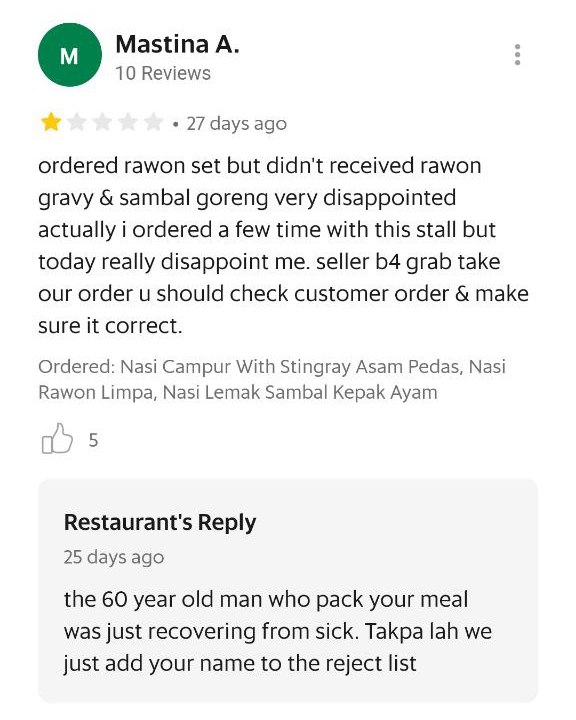Here is a cleaned-up and detailed caption for the image described:

---

The image displays a review section within a mobile app, characterized by a white background and a gray block section at the bottom, designated for restaurant supply. The review was left by Miss Mastina A, who has a total of 10 reviews. She rated the restaurant one star and left her review 27 days ago. In her feedback, Mastina expressed her disappointment due to incorrect order fulfillment. She had ordered a Raiwan set but did not receive the Raiwan gravy and sambal goreng. This oversight was particularly frustrating for her as she had successfully ordered multiple times from the same vendor previously. Mastina elaborated that she had ordered various dishes, including nasi campur with stingray, asam pedas, nasi raiwan, limpa nasi, lemak, sambal, and kepak ayam, and urged the seller to verify orders before dispatch. Her review received five likes. In response, the restaurant explained that a 60-year-old man, who had recently recovered from an illness, was responsible for packing her meal. They mentioned that Mastina's name would be added to their reject list.